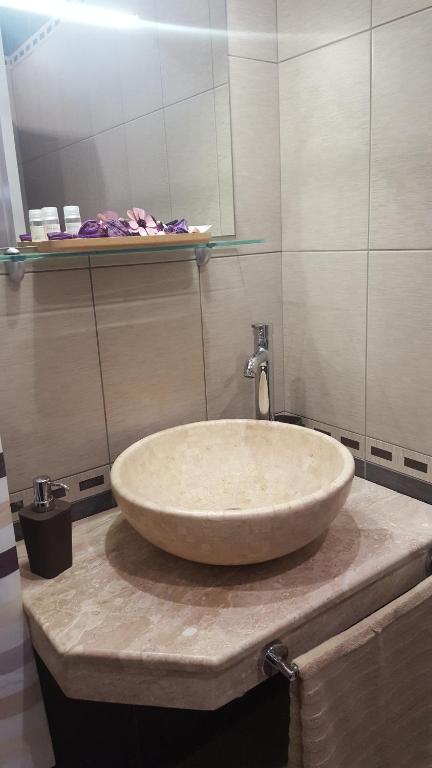This is a detailed photograph of a bathroom corner featuring a distinctive wash basin setup. The centerpiece of the image is a large, natural stone bowl sink in a light beige hue, sitting atop a medium brown granite countertop. A sleek, silver faucet emerges from the counter behind the bowl, enhancing its modern aesthetic. Hanging on the right side of the counter, you'll find a towel rack with a medium brown towel draped over it. The bathroom walls are adorned with large, tan, rectangular tiles that possess a matte, sandy finish, contributing to the rustic yet refined atmosphere.

Above the basin, there is a glass shelf mounted on the wall, holding a few essential oil vials, a little pink flower, and possibly some hand lotions. This glass shelf is positioned just beneath a rectangular mirror, which reflects light and adds depth to the space. Additionally, a dark brown or black soap dispenser is seen on the left side of the countertop. The countertop area is flanked by a curtain to the left, featuring white and brown stripes, which adds a touch of softness to the stony textures.